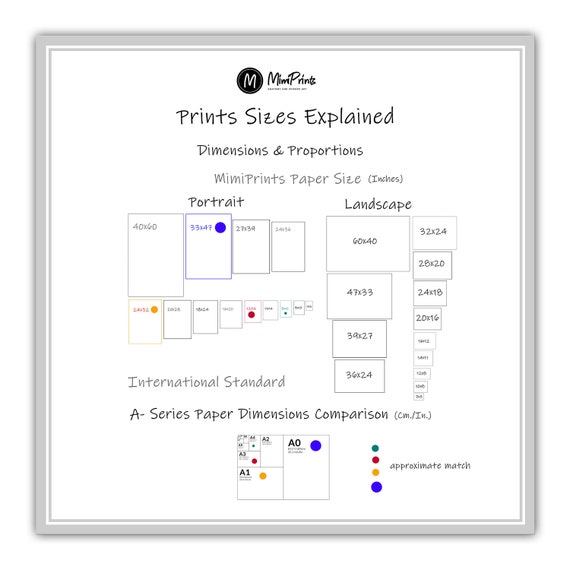The image depicts an informational chart with a grey border framing it, labeled with the logo of an 'M' encircled in black and titled "Mimiprints." The top of the chart explains "Mimiprints: print sizes explained, dimensions and properties," providing details in inches. It groups various portrait and landscape size samples separately, each labeled with dimensions. There are approximately 13 squares for both portrait and landscape, illustrating different size options. Below these, the chart includes an "international standard, A-series paper dimensions comparison" section, showing conversions from centimeters to inches with color-coded dots in blue, yellow, red, and green for easy reference.